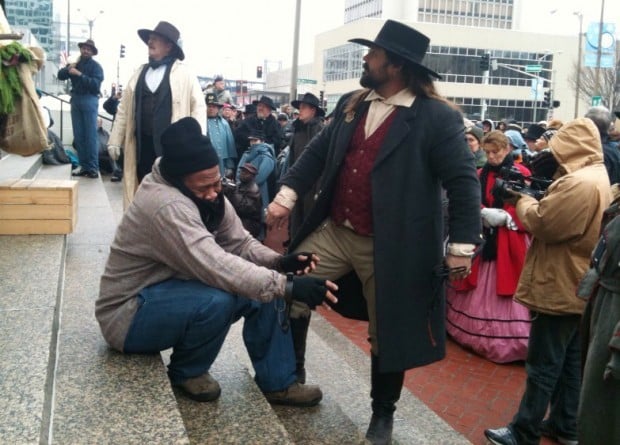The image captures a bustling reenactment event set in front of a grand city building with impressive marble steps leading to its entrance. The scene is lively with a large, captivated crowd gathered on the right side, intently watching the activity. Central to the image are three men dressed in period clothing reminiscent of the early 1800s, featuring long coats, red vests, and distinctive flat-brimmed black hats. They are all focused on something out of frame, adding an air of mystery. Adding to the historic theme, one individual is filming the event with a vintage 80s or 90s camcorder.

Contrasting the reenactors and the crowd, a man who appears to be homeless sits on the marble steps, dressed in a long-sleeved shirt, jeans, and a knitted black cap. He sports a significant black beard and mustache, seemingly indifferent to the surrounding excitement. The setting's architectural details include a red brick walkway and marble-patterned steps, adding to the richness of the scene.